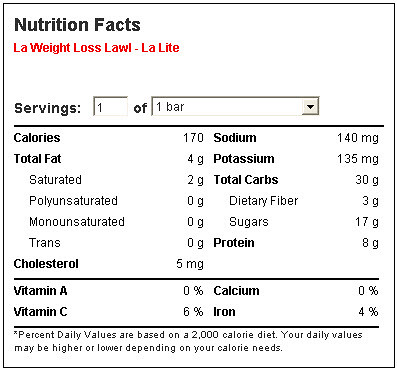The image displays a Nutrition Facts table in a digital format specifically designed for LA Weight Loss (marked as "LA Weight Loss, LAWL-LA Light" in red text). The table provides detailed nutritional information for a single serving size, indicated by a small box showing the number "1." Adjacent to this, there is a dropdown menu labeled "one bar" with a downward arrow for selection.

Below the serving information, the table covers various nutritional components, starting with calorie content, followed by a breakdown of total fat, cholesterol, sodium, potassium, total carbohydrates, and protein. Further down, there is a section detailing the amounts of Vitamin A, Vitamin C, calcium, and iron. At the bottom of the Nutrition Facts table, a disclaimer notes that the % Daily Values are based on a 2,000 calorie diet, with an additional statement indicating that individual daily values may vary depending on specific calorie needs.